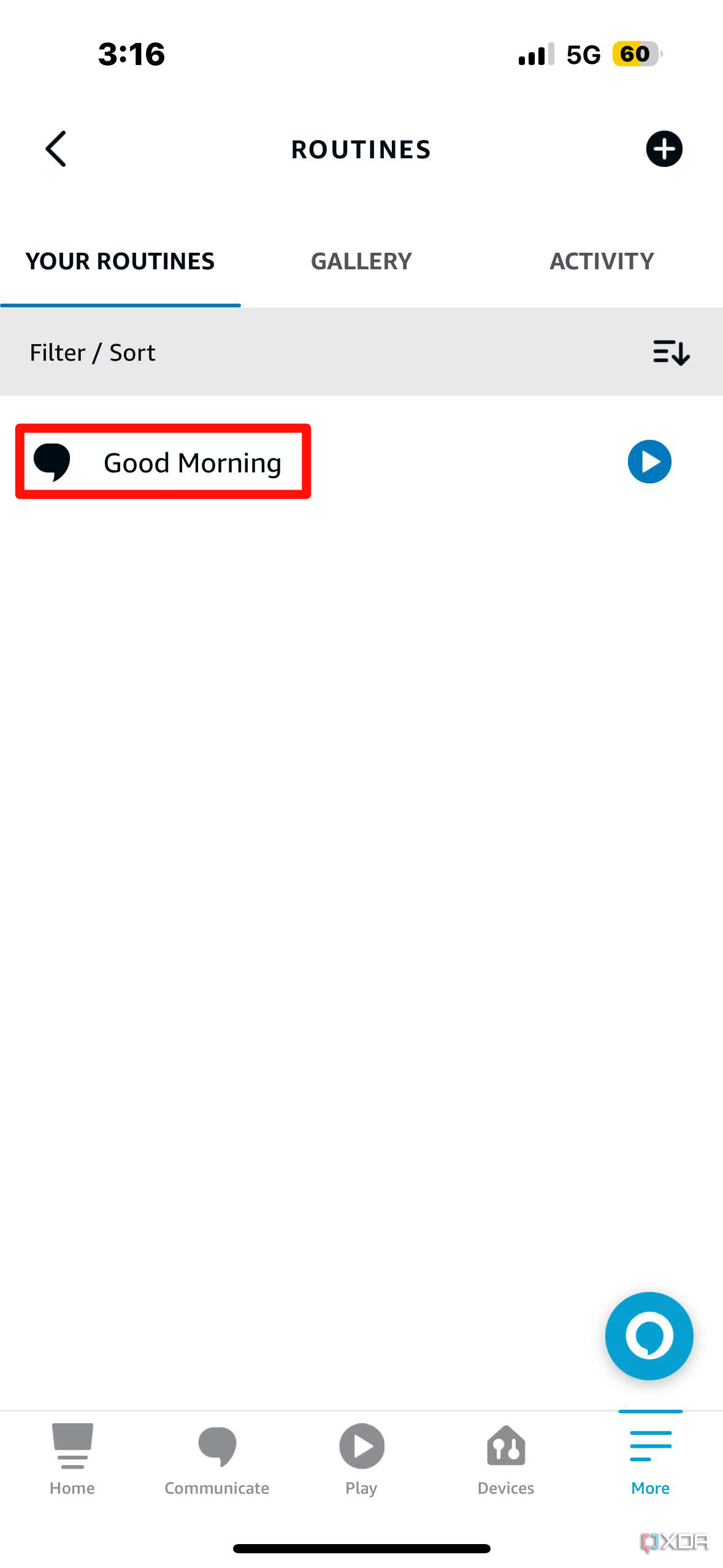The top left-hand corner of the image displays the number "316". On the top right-hand corner, there are four ascending bars indicating signal strength; the first three bars are black, and the fourth bar is gray. Next to them, it says "5G". Below, there is a button, half yellow and half gray, with "60" written on it. An arrow pointing to the left is labeled "routines".

Adjacent to this arrow is a black circle containing a white plus sign, followed by the text "your routines" underlined in blue. Below this, there are the words "gallery" and "activity". A gray rectangle labeled "filler/sort" is situated nearby. Additionally, there are lines with a downward-pointing arrow beside them.

A red-outlined rectangle resembling a speech bubble contains the message "good morning". A blue circle with a white right-pointing triangle is present as well. The lower portion of the image has significant blank space.

On the right-hand side of the image, there is a blue circle enclosing a smaller white circle, with a blue speech bubble-like shape protruding from it, underlined in blue. Below this underlined blue text, a gray line spans the width of the image.

Towards the bottom, there is a rectangular icon with two lines beneath it labeled "home". A speech bubble icon labeled "communicate" appears next. A gray circle with a right-pointing triangle is labeled "play". An icon of a house with two indiscernible items inside has "devices" written below it.

At the bottom right, three horizontal blue lines are stacked, with the third line being shorter. Below these lines, "more" is written. Lastly, a black line runs along the very bottom of the image.